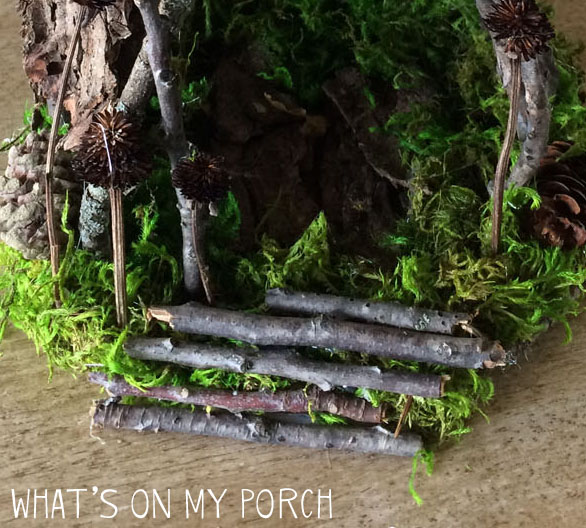The photograph depicts the base of what appears to be a large, weathered tree that has a hollowed-out section. The textured surface, which could be mistaken for stone, adds to the aged and rugged appearance of the tree. Clusters of green moss adorn the hollow, suggesting an undisturbed natural environment. In front of the tree, a small bundle of sticks lies scattered. At the bottom of the image, white text reads, "What's on my porch?" However, the image itself does not provide any clear indication of what is on the porch, leaving the question unanswered.